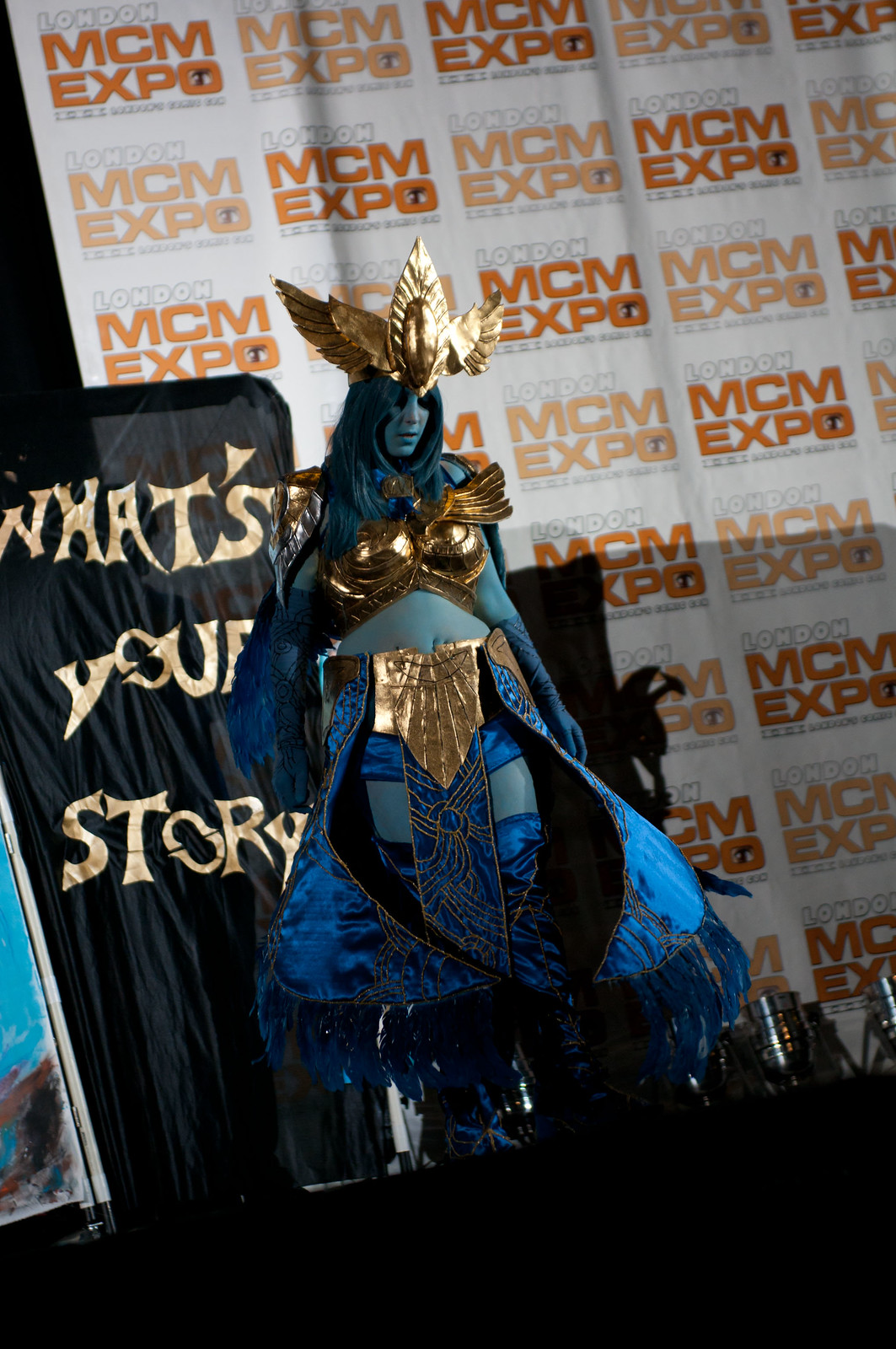The photograph captures a young woman in an elaborately detailed cosplay costume, standing on a dark stage. She is the central focus of the portrait-oriented image. She is dressed as a bird-like character, showcasing a gold beak and eyes, and adorned with vibrant bird-like feathers. Her outfit consists of a blue skirt that flares outward, complemented by a gold band around her waist, and a golden breastplate. She also wears a distinctive gold crown with gold wings. The woman’s striking blue makeup and hair enhance her fantastical appearance. To her left, a black sign with gold lettering reads, "What's Your Story?" Behind her, in the background, is a white backdrop featuring an orange "MCM Expo" logo. The image is taken at an angle, from the bottom right to the top left, providing a dynamic perspective of the scene. Additionally, the bottom right-hand corner of a framed drawing is partially visible to the left of the sign, adding an element of artistic intrigue to the setting.